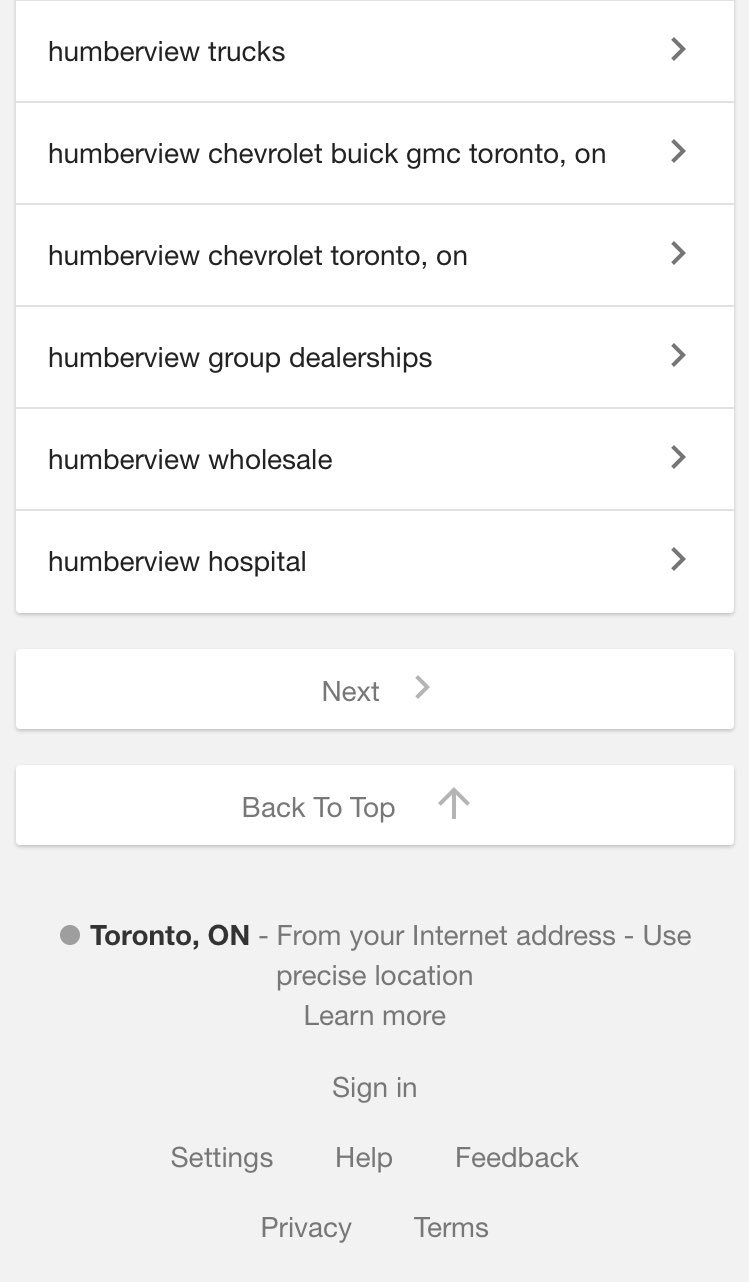The image features a white background with a series of elements arranged in a structured format. At the top, bold black text reads "Humber View Trucks" with a right-pointing arrow on the far right. Beneath this, a fine gray line separates the top element from the next. The text "Humber View Chevrolet Buick GMC, Toronto, ON" appears next, accompanied by a small gray right-pointing arrow. Another fine gray line follows.

Next, the text reads "Humber View Chevrolet, Toronto, ON" with a similar right-pointing gray arrow and fine gray line beneath. This structure continues with "Humber View Group Dealerships" followed by the arrow and fine gray line, then "Humber View Wholesale" with the same arrow and line.

The sequence continues with "Humber View Hospital" along with another gray arrow and line. The pattern is interrupted by a white space and another white banner in the middle, which contains the word "Next" and a small gray arrow pointing right.

A similar pattern follows with another white space and white banner featuring the text "Back to top" in gray with an upward-pointing arrow. 

At the bottom, the image is shaded gray. It displays the text "Toronto, ON" on the left side along with a gray button. The text "— From your internet address — Use precise location, learn more" follows, along with a "Sign In" button. Below this, there are options labeled "Settings," "Help," and "Feedback," followed by "Privacy" and "Terms."